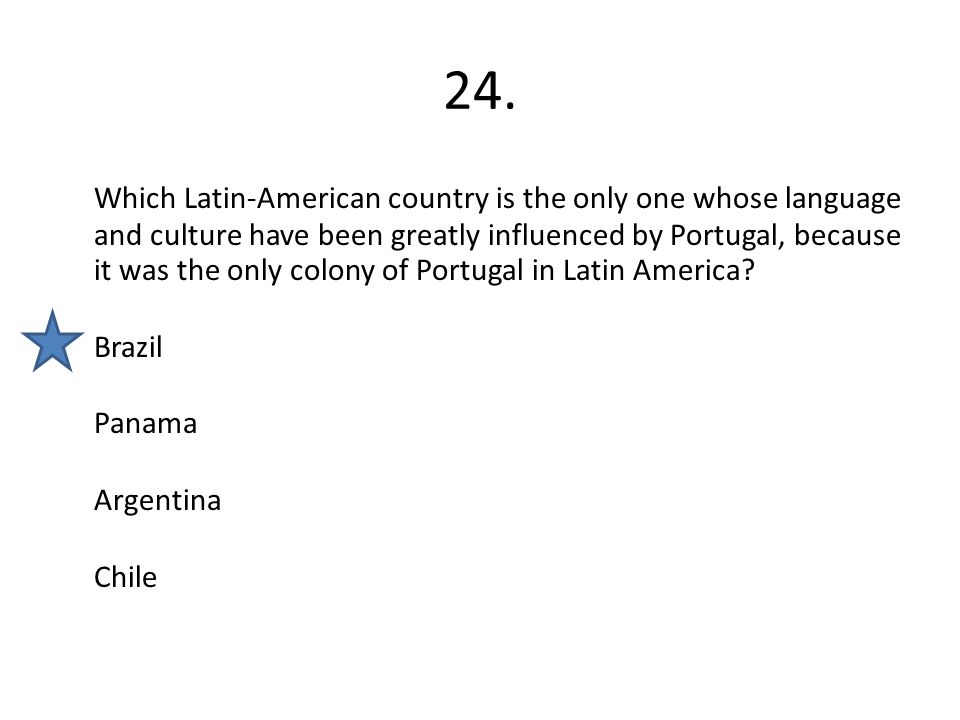The image depicts a quiz screen displaying a multiple-choice question about Latin American countries. At the top of the screen is the number "24," followed by a period, in the largest font on the screen. Below this, the question reads: "Which Latin American country is the only one whose language and culture have been greatly influenced by Portugal because it was the only colony of Portugal in Latin America?" 

Four answer choices are listed vertically along the left side of the image: Brazil, Panama, Argentina, and Chile, each separated by a small space. A blue star with a navy-edged, slightly two-dimensional or three-dimensional appearance is positioned next to the word "Brazil," indicating it as the correct answer. The font size of the answer choices appears slightly larger than the font used for the question text.